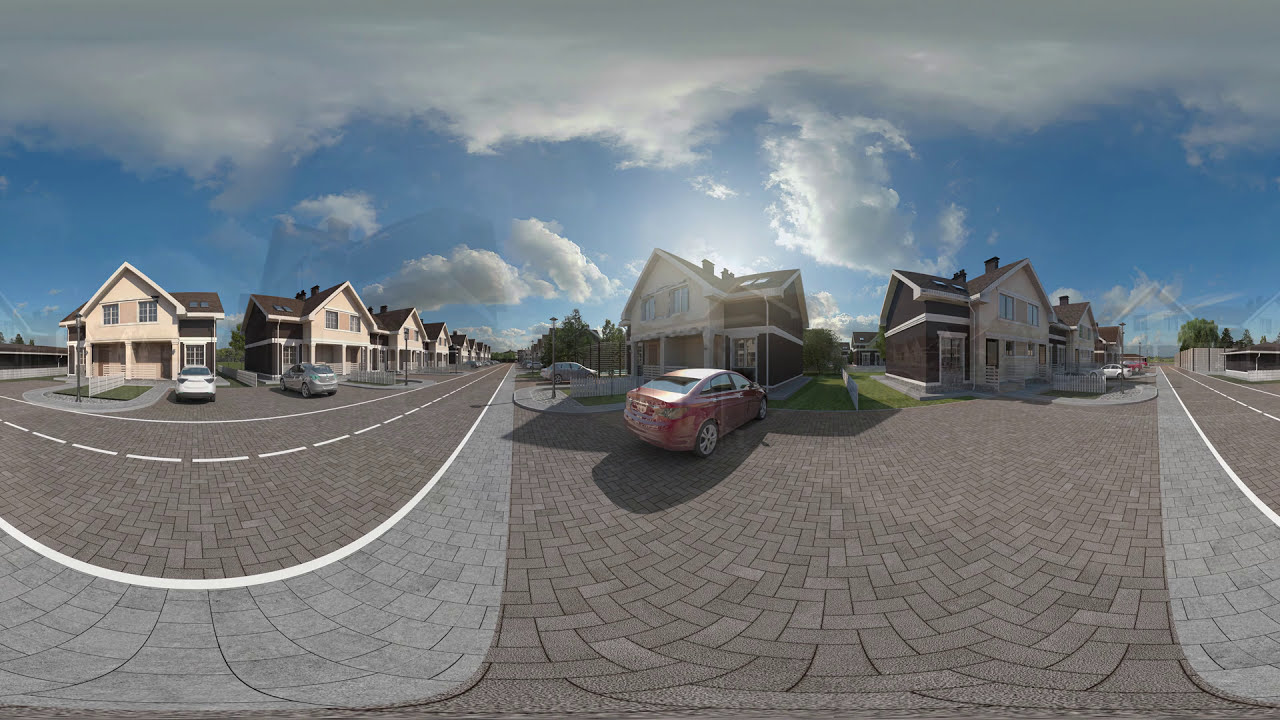The image captures a picturesque residential neighborhood under a bright daytime sky with scattered white clouds, some of which are highlighted by the sunlight shining from behind a two-story house in the center. The neighborhood features distinct and decorative red brick streets, detailed with a dotted white line in the center and solid lines on the sides, curving gracefully around the houses. The houses, mostly moderate in size and similar in style, line both sides of the streets. On the left, the road curves and leads out of the frame, flanked by homes with small trees interspersed. In the middle of the image, in front of a house with a combination of brick and lighter siding, a small red four-door sedan is parked. Another street goes straight towards the background on the right, emerging from a parking area and disappearing into the distance. The overall cleanliness and uniformity of the houses and streets give the scene a pristine and almost cinematic quality.